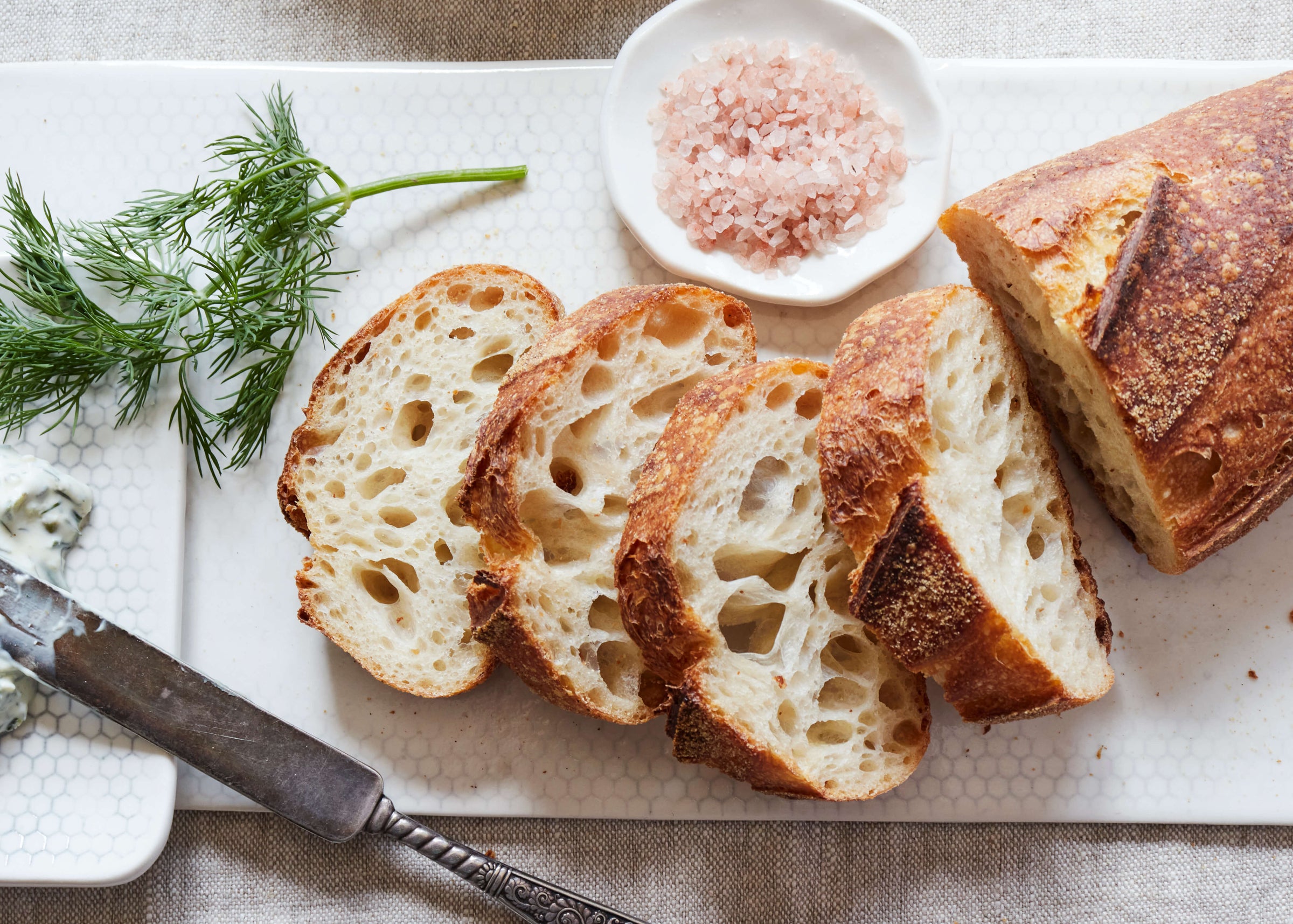The image features an appetizing spread presented on a flat white stoneware plate with a subtle circular pattern. Central to the arrangement is a freshly baked loaf of bread, likely a French loaf or baguette, characterized by its crispy, brown-orange crust and airy, hole-filled white interior. Four slices of the bread are cut and arranged neatly, leaning against each other, with the remaining part of the loaf positioned to the right. Above the slices, there is a small, slightly uneven white bowl containing pinkish-white Himalayan salt crystals. To the left of the bread slices lies a sprig of green herb, possibly dill, adding a touch of freshness to the presentation. Partially visible at the bottom is an ornate butter knife with a silver blade and a wooden handle, resting on the plate with remnants of a white spread, likely intended for the bread. The entire setup rests on a table or tablecloth of a grayish color with fabric striping, enhancing the rustic elegance of the display.